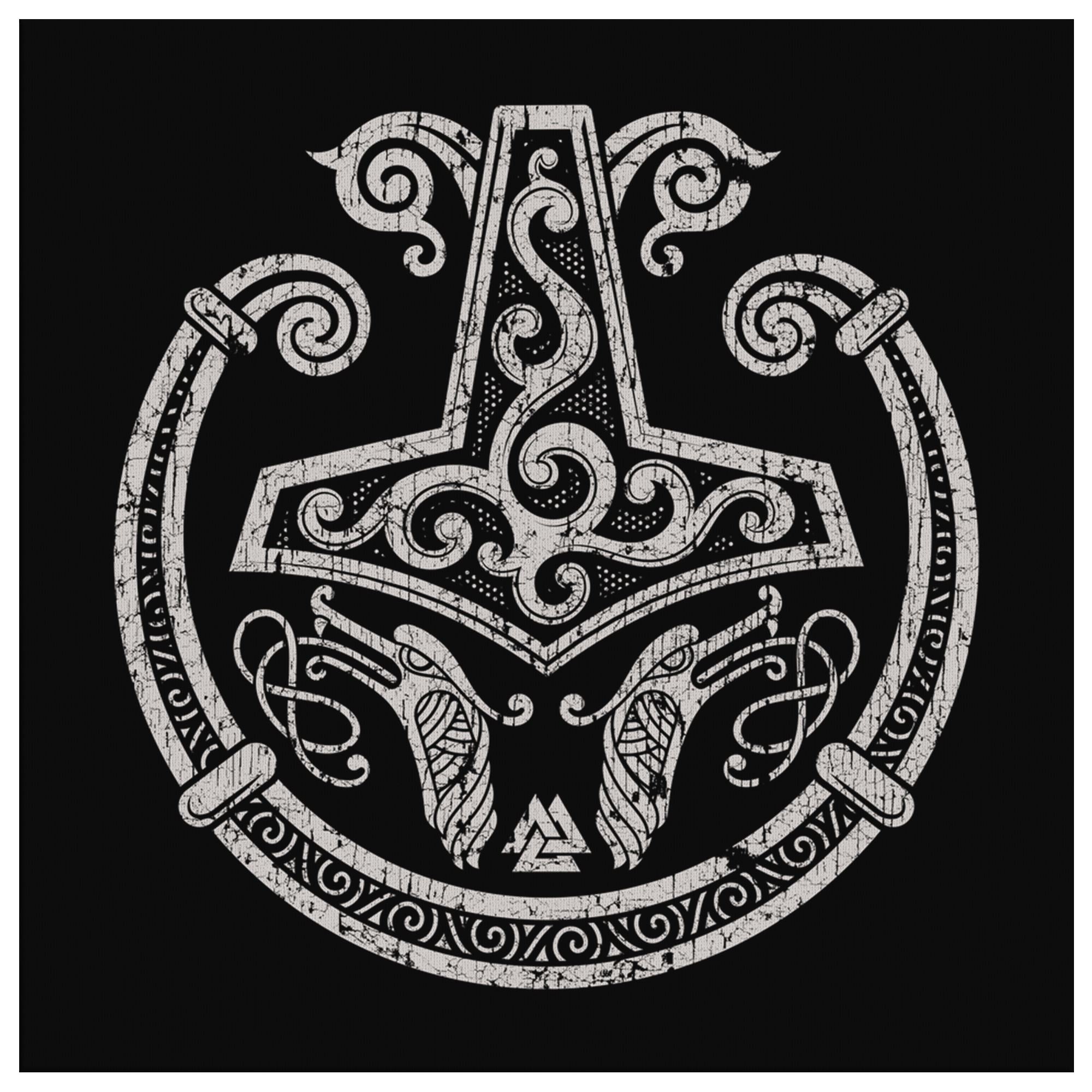The image captures a close-up view of a metallic, emblematic object set against an all-black background. The bottom section of the emblem is characterized by a semi-circular shape with intricate wavy lines and a border resembling a nearly full circle. This border is segmented by lines that divide the semi-circle into distinct sections. Above this, the design features two curved forms that resemble abstract fists, lacking detailed fingers and swirling towards the center.

In the middle of the emblem lies a design that closely resembles a pilgrim's hat, adorned with intricate, wavy lines along the top of its crown. Between the semi-circular border and the pilgrim hat motif, there are two dragon heads facing away from each other, one looking left and the other right. Nestled between these dragon heads are three interconnected triangles, positioned just behind the heads, adding a geometric touch to the overall intricate design.